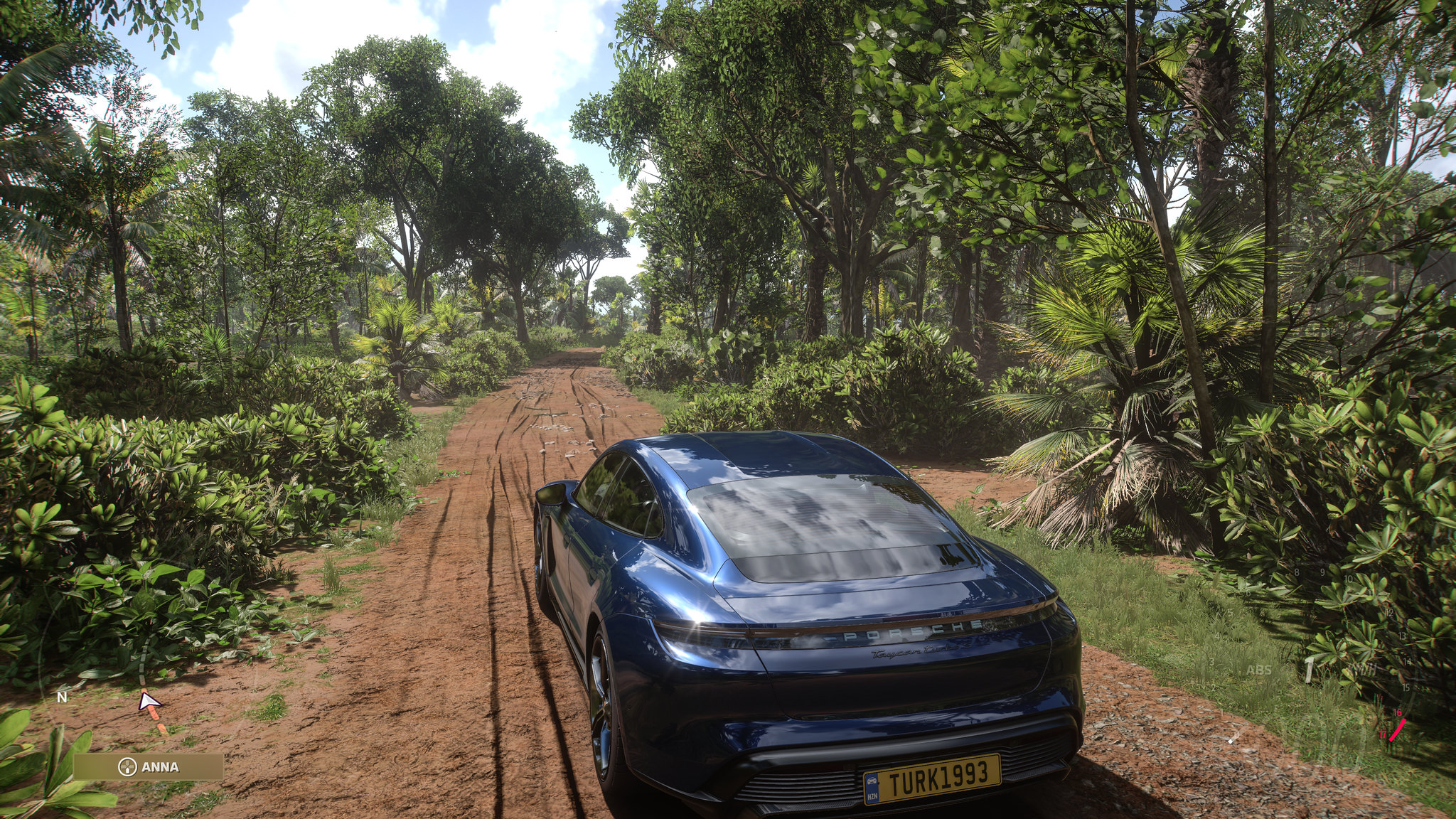The image showcases the rear view of a striking blue Porsche sports car with a small yellow license plate reading "Turk 1993" at the bottom. The car appears to be on a well-maintained, flat dirt road, likely part of a private property. The surrounding scenery includes an array of lush greenery, shrubs, and a variety of trees, such as palm trees and other types, lining both sides of the path. On the left side, there's a path of plants and a tiny box labeled "Anna" with a drone-dotted line and a white arrow pointing ahead. The sky overhead is a vibrant blue, spotted with fluffy white clouds, adding to the overall idyllic, almost surreal quality of the scene.